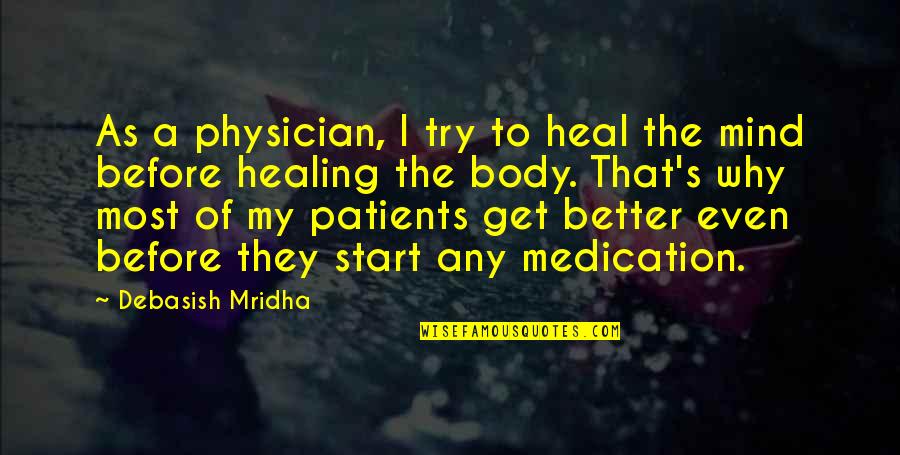The image is a graphic featuring a prominent quote by Debashish Mridha: "As a physician, I try to heal the mind before healing the body. That's why most of my patients get better even before they start any medication." The quote is centered in bright yellow sans-serif text, creating a sharp contrast against the dark background. The background image, which is heavily overlaid with a black filter, appears to feature splashing water, with possible elements like a red star-shaped item or a flower, but these details remain indistinct due to the overlay. The background also shows highlights where light hits the water, creating scattered reflective spots. Beneath the quote, there is a small bright yellow rectangle containing the black text "wisefamousquotes.com." The overall design suggests that this image is intended for sharing online, likely as an inspirational meme.